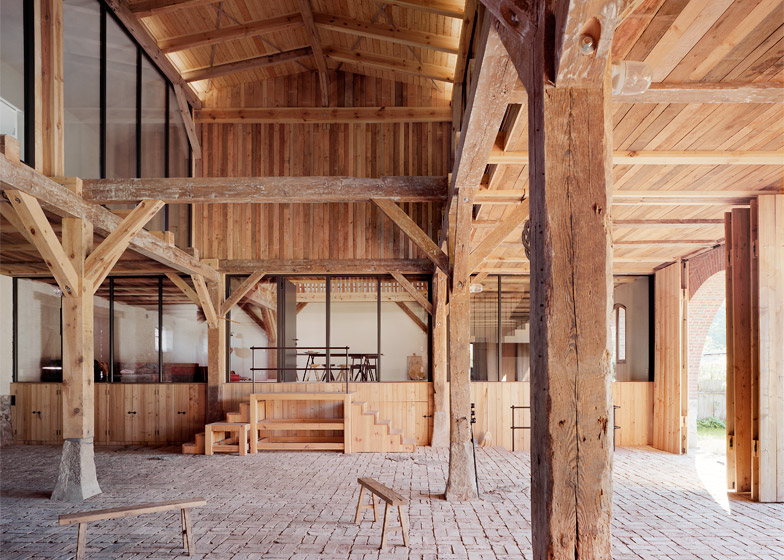A meticulously remodeled barn interior showcases a harmonious blend of rustic charm and modern functionality. Aged vertical and cross beams hint at the barn's storied past, while the expansive, open center and cathedral-like ceiling evoke a grand sense of space. Large glass partitions delineate separate areas, suggesting a versatile future use as office spaces or perhaps a sophisticated winery. The design marries the rustic essence of a high-end garage with the elegance of a professional office environment. The structure features a striking post-and-beam construction with an abundance of reclaimed wood, creating a warm and inviting atmosphere. The floor is beautifully paved, and the walls are equipped with sliding and roll-open doors, enhancing accessibility and fostering a seamless indoor-outdoor flow. This remarkable transformation highlights the barn's enduring architectural beauty and its potential for diverse, modern applications.